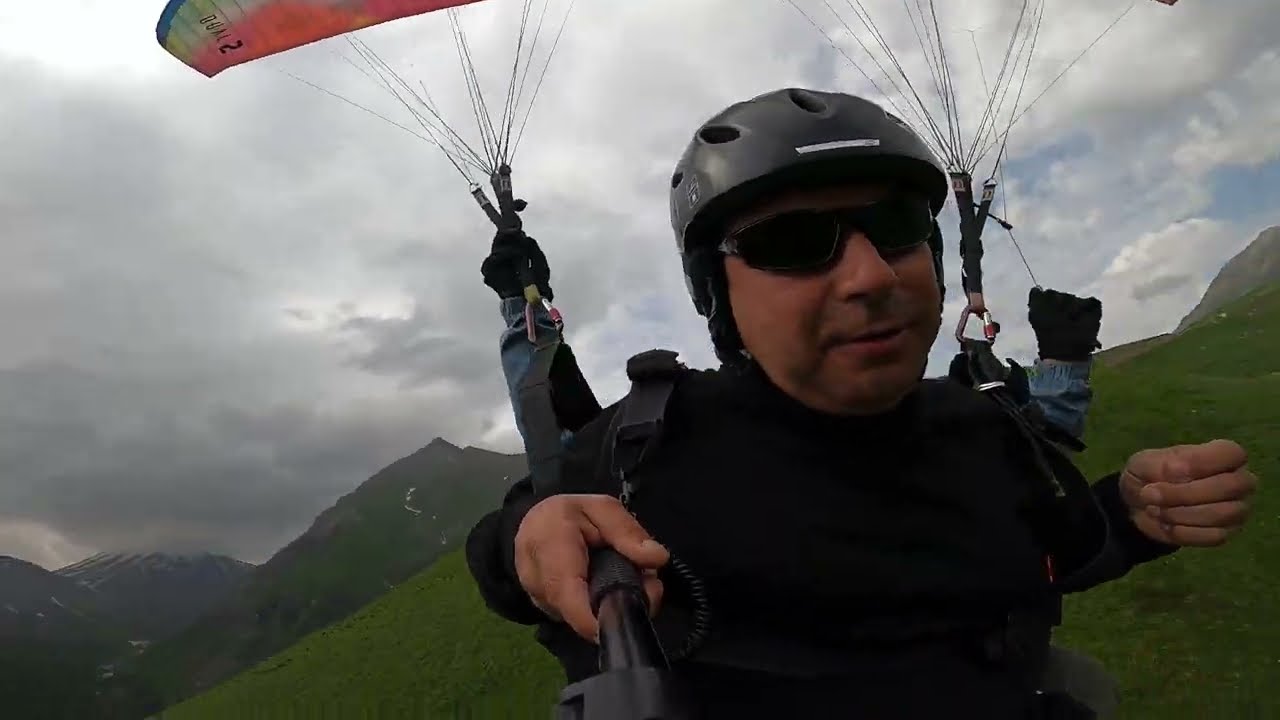In this dynamic selfie of a man paragliding, he captures the breathtaking combination of mountainous terrain and a dramatic sky. The man, dressed in all black with a helmet, long-sleeved jacket, harness, and dark sunglasses, exudes an air of adventurous readiness. He wields a black selfie stick that frames the shot perfectly. Suspended and gliding, his colorful parachute—adorned with shades of orange, white, yellow, blue, and marked with black numbers—stands out vividly against the backdrop. The sky behind him is a mix of dark gray and light blue, heavily overcast with a hint of blue peeking through the clouds, suggesting an impending storm. The mountainous landscape below features snow-capped peaks and lush green flatlands, adding to the image’s striking contrasts. This self-portrait, possibly taken with a smartphone given its slight distortion, encapsulates a moment of serene thrill, with the man’s poised posture and the expansive, cloud-filled sky hinting at both tranquility and the rush of adrenaline.